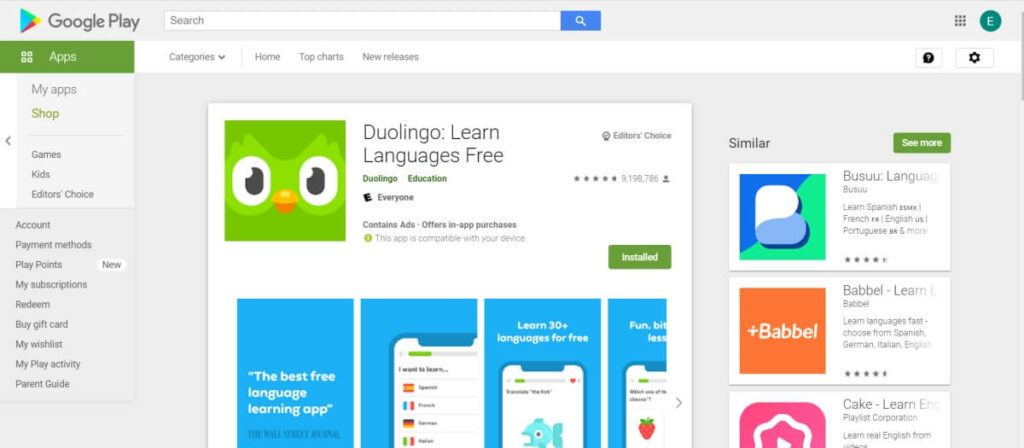The image is a screenshot from a Google Play webpage displayed on a computer screen. At the top of the page, there is a search bar, which ends with a small blue box containing a magnifying glass icon, signifying the search function. To the right of the search bar, there is a grid-like cube icon composed of multiple smaller squares, next to which is a large capital "E" within a green circle, likely representing a user profile or a specific section.

On the left-hand side of the webpage, there is a navigational menu. It features several categories:
- Apps (highlighted and expanded to show "My Apps" in focus)
- Shop (highlighted in green)
- Games
- Kids
- Editor's Choice.

Further down the menu, additional options are listed, including:
- Account
- Payment Methods
- Play Points (marked as a new feature)
- My Subscriptions
- Redeem
- Buy Gift Card
- My Wishlist
- My Play Activity
- Parent Guide.

Central to the image, prominently displayed, is a green square featuring an owl's face, representing the app Duolingo with the caption "Learn Languages Free" beside it. Below this, there are details indicating the app contains ads and offers in-app purchases, along with a green rectangle that reads "Installed." Surrounding this main area are other images and icons related to various apps and functions on the Google Play store, offering additional clickable options.